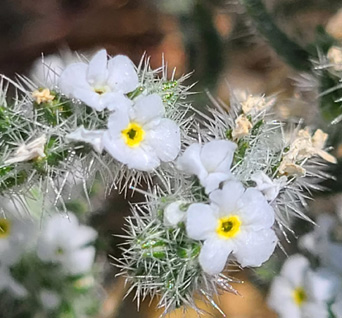A vivid, close-up color photograph captures the intricate details of a cactus. The green flesh of the cactus is prominently displayed, adorned with numerous sharp spines. Adding to its natural beauty, several small white flowers are in bloom, each with five delicate petals. At the center of each flower, a yellow circle encircles a smaller dark circle, creating a striking contrast against the white petals. The background, although out of focus, reveals an array of additional cacti, also adorned with similar blossoms, enhancing the richness of the scene. There are no human figures, animals, or man-made objects present, allowing the natural splendor of the cacti and their blooms to take center stage.